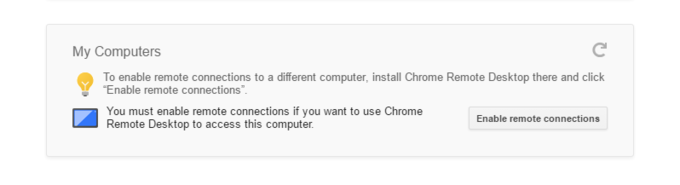The photograph depicts a computer screen displaying a notification message. The message is presented within a long, horizontal rectangle featuring a white background. In the upper left corner, dark bluish-purple text reads, "My Computer." Directly below this text, there is an icon of a light bulb, colored with a yellow or gold top and a blue bottom.

The message following the light bulb icon states: "To enable remote connections to a different computer, install Chrome Remote Desktop there and click 'Enable Remote Connections.'"

Beneath this instruction, another icon appears. This icon is a small rectangle divided diagonally, with the lower triangle in dark blue and the upper triangle in light blue. Accompanying this icon, the text states: "You must enable remote connections if you want to use Chrome Remote Desktop to access this computer."

On the right side of the notification is a button with a white background labeled "Enable Remote Connections." In the upper right-hand corner of the screen, a refresh symbol, consisting of a circular arrow, is also visible.